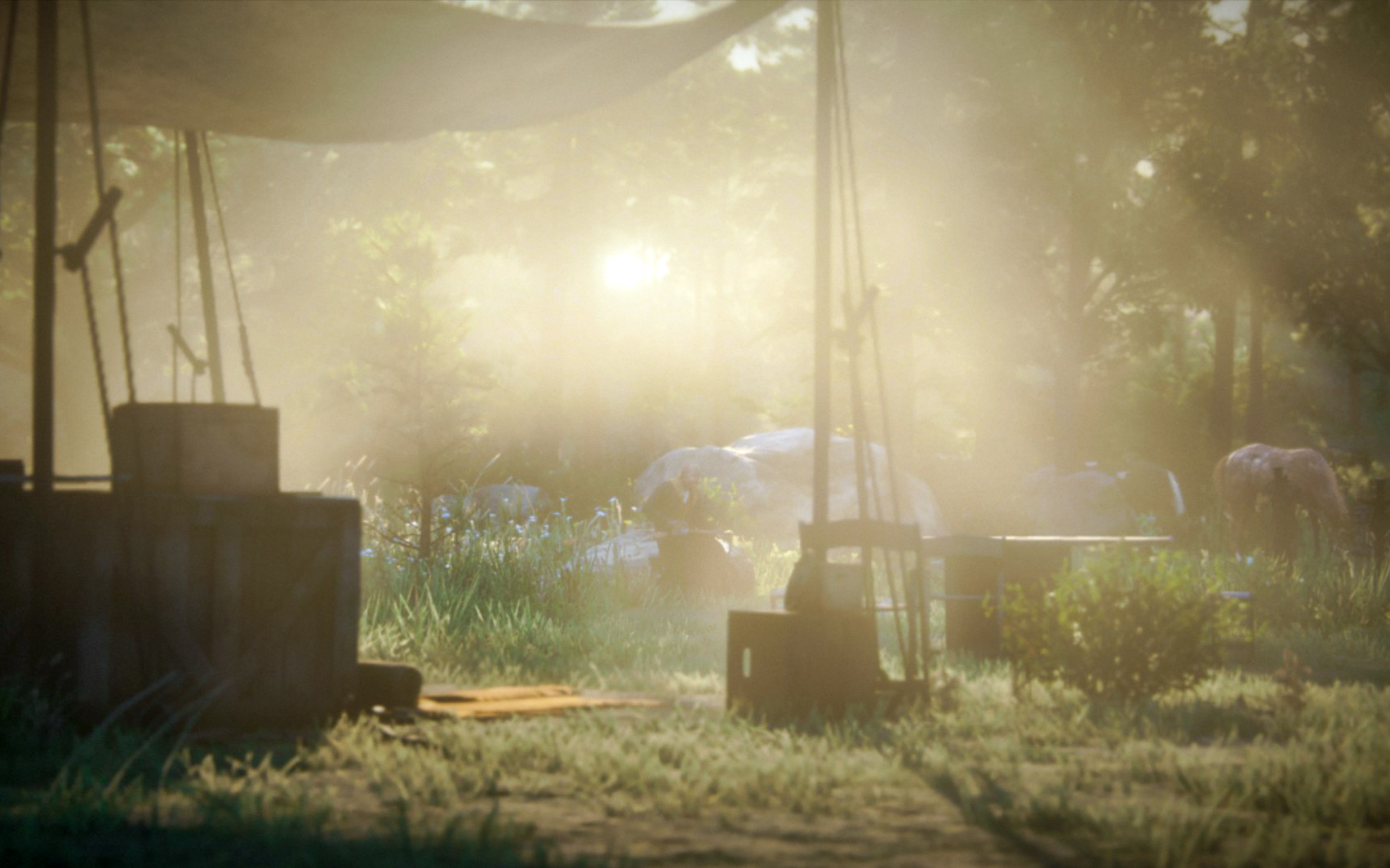This color photograph captures an early morning scene at what appears to be a campsite, possibly a traveling circus. There is a noticeable glare from the sunlight streaming through the trees, creating a misty and slightly obscured view. In the background and towards the very right, an elephant can be seen, though it is distant and somewhat small, partially hidden by the trees. The campsite features several tents, including a prominent white one among other smaller structures. There's a large open tent held up by poles and ropes, underneath which lies a tarp sheltering numerous brown or tan boxes, possibly wooden crates.

The foreground details include a combination of grass and patches of dirt, with a bush situated in the lower right corner. Near the tarp, there are additional structures and items: boxes, possibly made of wood or cardboard, a couple of chairs, and some ropes and stakes securing the tent setup. The sunbeams filtering through wash out parts of the trees behind, while casting light that highlights the greens and the scene's morning haze. A few tents and what might be a man sitting on a rock are also discernible in the midground. The overall setting is amidst a grassy field surrounded by trees, evoking the organized yet transient nature of a circus or large outdoor gathering.